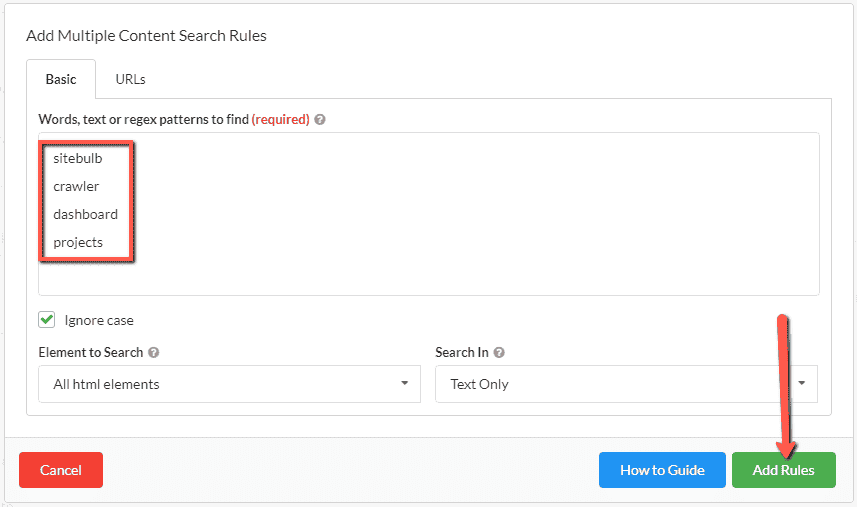Screenshot of a content search interface:

The image displays a user interface for adding content search rules, bordered in light gray. At the top, there's a heading in dark gray or black that reads "Add Multiple Content Search Rules." Below this, two options are presented: "Basic" and "URLs," with "Basic" selected. A red, parenthetical note beside the input field states "(Required)," indicating that text, words, or regex patterns need to be specified. A question mark icon is present next to the required input field.

Highlighted in a red-bordered rectangle, the text "Sitebulb Crawler Dashboard Projects" is shown prominently. Below this, there’s an option labeled "Ignore case," accompanied by a green check-marked box. Following that, the interface asks for "Element to search" and "Search in," both featuring question mark icons for additional help.

Underneath these options, there are two drop-down search boxes, one labeled "All HTML elements" and the other "Text only," each with a downward arrow indicating additional selection options.

At the bottom, the interface presents three buttons: a red triangle labeled "Cancel" on the bottom left, a blue rectangle labeled "How to Guide" in the middle, and a green rectangle labeled "Add Rules" on the bottom right. Additionally, a red arrow graphic points downward towards the "Add Rules" button, likely emphasizing its importance.